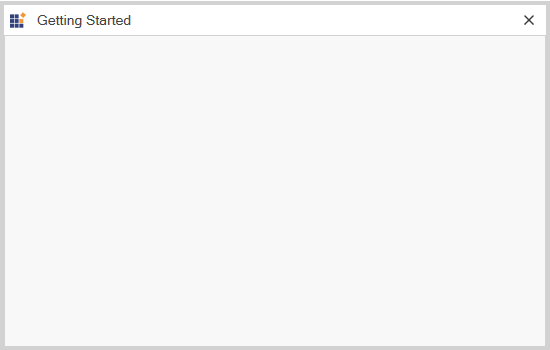Caption: 

The image showcases a minimalist window titled "Getting Started," prominently displayed with a cohesive color scheme. In the upper left corner, a small icon consisting of a 3x3 grid of squares is visible. The majority of the squares are blue, however, the top-right section of the grid appears to be in a state of transition with two orange squares either assembling or disassembling, adding a dynamic element to the otherwise static image. The background of the window is a blank expanse of gray, suggesting either incomplete development or a placeholder for future content. To the top right of the window, an 'X' button serves as an exit option. The entire window is framed by a slightly darker gray border, providing a subtle yet distinct boundary.